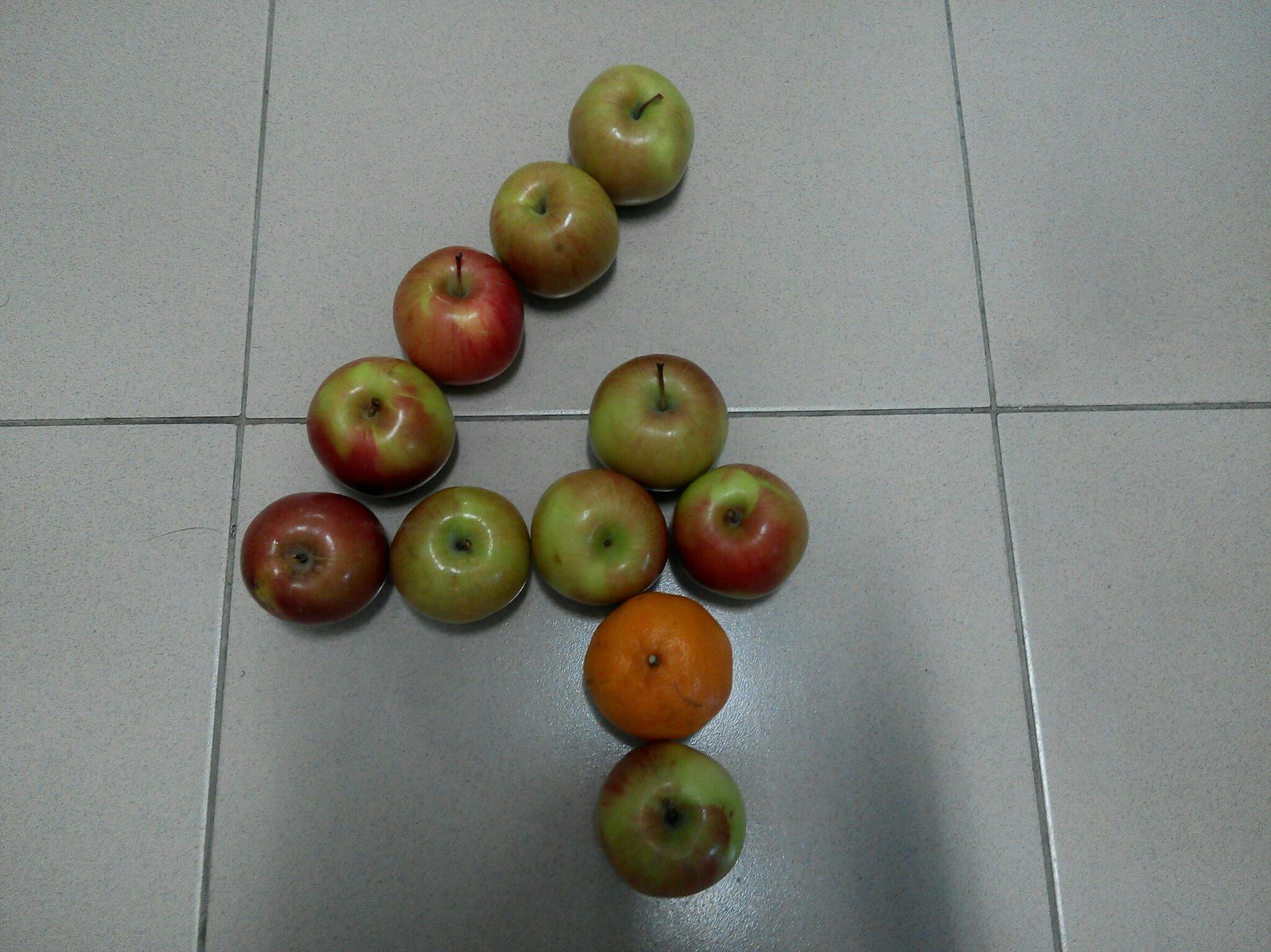The photograph features a clean, white tiled floor with gray grout, captured from above. Arranged in the center are about a dozen apples forming the shape of the number four, which has an open-back style resembling an arrow pointing left with a line underneath. Most apples exhibit a mix of light green and red hues, indicative of Pink Lady apples, known for their sweetness. Among them, towards the bottom of the formation, sits a single navel orange with a couple of bruises. Notably, the apple beneath the orange appears to be beginning to rot from the center outward. There is no text or metadata indicating the date or location of the photograph, implying it was taken indoors.